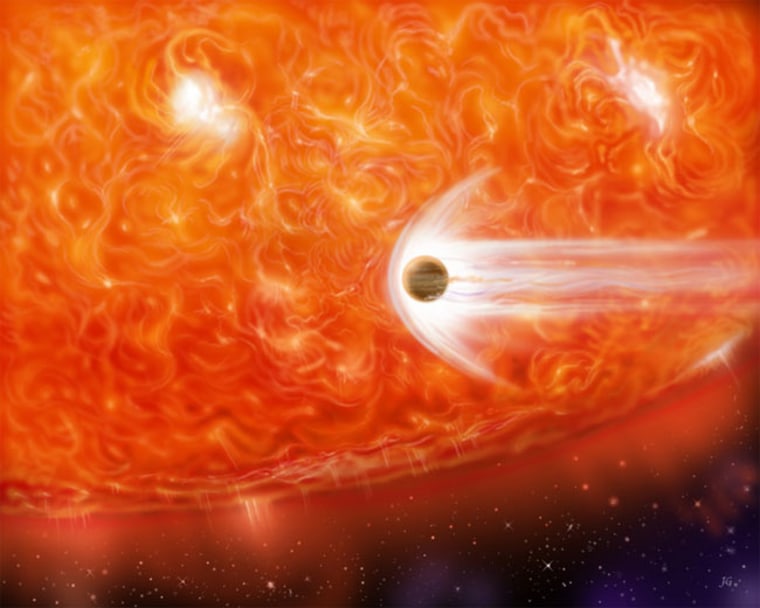The photograph, likely captured by the Hubble Telescope or digitally created, features a vivid and dynamic scene in outer space. Dominating the top half of the image is the intense and fiery surface of the sun, characterized by bright orange and red swirls interspersed with yellowish-white firestorms. In the upper left portion, a prominent solar flare about three-quarters of an inch in diameter emanates from the sun's surface, casting a gleaming white light. Another, slightly smaller, oval-shaped flare can be seen in the upper right of the photograph.

Centrally located in the image, there is a small, tan and dark brown planet—potentially Mercury—seemingly in motion due to the bright white arc of light enveloping it and the streaks of white light trailing behind it, resembling the vapor trail of a jet breaking the sound barrier. This effect gives the impression that the planet is streaking across the surface of the sun.

The bottom of the photograph transitions into the blackness of space, with small, scattered white stars punctuating the dark blue expanse. The overall composition blends the glowing intensity of the solar activity with the serene backdrop of the cosmos, creating a striking and dynamic portrayal of both celestial bodies and the void they inhabit.